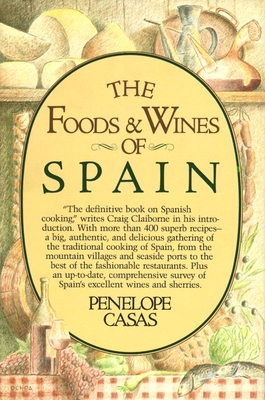The front cover of this book, "The Foods and Wines of Spain" by Penelope Casas, features a large vertical oval at its center. Within the oval, the title is prominently displayed in brown and black text, followed by an introduction by Craig Claiborne, which praises the book as "the definitive book on Spanish cooking." It boasts more than 400 recipes, offering an authentic and delicious array of traditional Spanish cuisine, from mountain villages and seaside ports to fashionable restaurants, along with an in-depth survey of Spain's wines and sherries. The author's name, Penelope Casas, is printed at the bottom in black. 

Surrounding the oval is an intricate illustration of various foods. At the top, there is a tan wooden shelf holding bread on the left and containers of liquids on the right, creating a rustic kitchen ambiance against a beige, wood-paneled wall. Below, a wine bottle and a crystal glass, half-filled with wine, are accompanied by a bunch of grapes. On the right side, some fish, and on the left, scattered vegetables, add to the culinary theme. The overall background suggests a cozy dining setting, emphasizing the book’s focus on rich, traditional Spanish gastronomy.